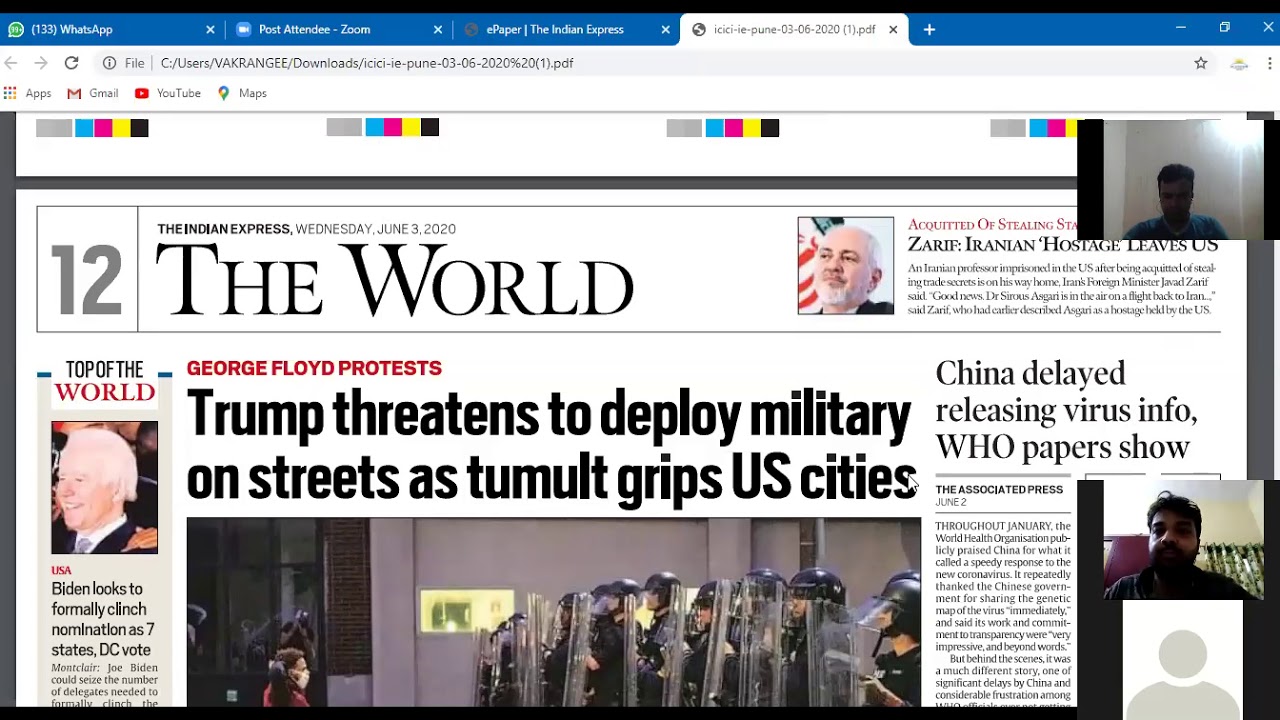This image depicts an open web browser on a computer screen. The browser's top bar is a plain black strip devoid of any visible icons or text. Four tabs are open within the browser. The first tab is for WhatsApp, the second is titled "Post Attendee Zoom," the third tab's title is partially obscured but includes the word "express," and the fourth tab, which is currently active, displays a digital copy of an Indian Express newspaper dated Wednesday, June 3, 2020.

The browser URL indicates that this newspaper is accessed from a local file path: C:\Users\Fakranji\Downloads, suggesting the PDF has been downloaded. The newspaper, titled "The World," features several headlines and images. To the right of the title, a headline reads, "Zarif, Iranian hostage leaves us, acquitted of stealing," partially obscured by a square overlay with someone's face.

Below the main article, there's a column titled "Top of the World" with a photograph of Joe Biden alongside related text. Adjacent to this column, another headline covers the George Floyd protests, stating, "Trump threatens to deploy military on streets as tumult grips U.S. cities," accompanied by a relevant image. On the far right, a headline declares, "China Delayed Releasing Virus Info, WHO Papers Show." Below this, another inset shows an individual’s face, possibly indicating a live video feed or additional commentary.

This image captures a snapshot of contemporary headlines and the digital interface through which many now consume news.